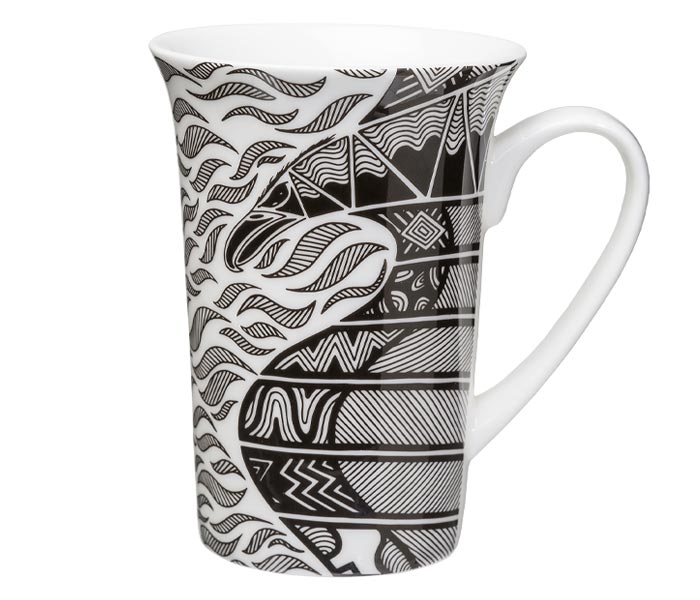This photograph captures a vertically-oriented, ceramic mug that stands taller than a typical coffee mug. The mug features a distinctive black-and-white design that covers its entire exterior. The design is split into two parts by a curved 'S' shape. The left side is predominantly white, adorned with black and white swirls and leaf-shaped patterns. The right side contrasts sharply, dominated by a fierce-looking bird head, resembling an eagle or hawk. This bird has slanted eyes that contribute to an angry expression, a scowling beak, and is segmented into geometric shapes and lines. The mug's interior and handle are white, further emphasizing the striking exterior design. The background of the image is pure white, keeping the focus solely on the intricate and abstract beauty of the mug.